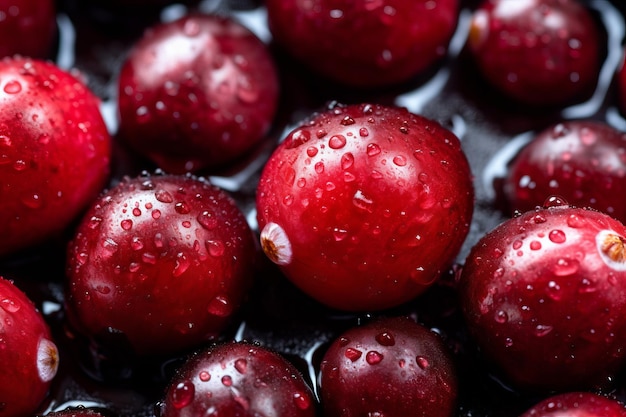The photograph is a meticulously detailed artistic close-up of approximately a dozen fresh cranberries, arrayed on what seems to be a black surface. Capturing every intricate feature, the image showcases the cranberries with droplets of moisture, suggesting they were recently washed or rained upon. The cranberries, in a variety of sizes from small to large, exhibit a beautiful ripe crimson red hue with light reflections that seem to originate from an indoor source, possibly a window, rather than direct sunlight. This touch of light adds a gleam to each berry, enhancing their vibrant and glossy appearance, as if they are being prepped for a culinary use.